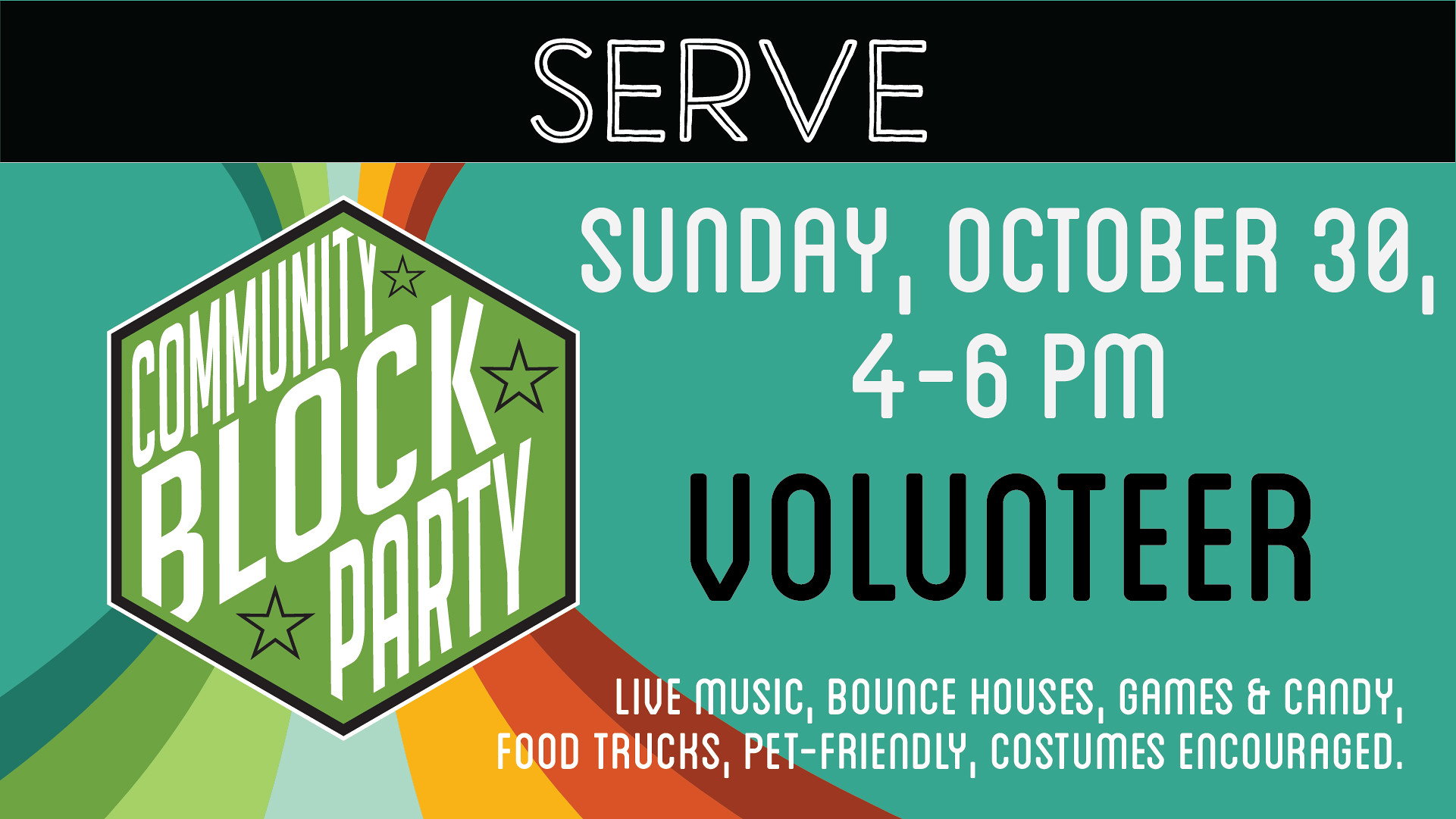The image features a vibrant green background with a prominent black stripe along the top, where the word "SERVE" is displayed in bold, white capital letters. Below this, on the left side of the green background, there's a green hexagon outlined with white. Inside the hexagon, it reads "Community Block Rock Party" with three black stars accompanying the text, all set against the colorful backdrop of a rainbow. On the right side, white text provides event details: "Sunday, October 30th, 4 to 6 p.m." followed by "Volunteer" in black. Further information includes enticing activities in white letters: "Live Music, Bounce Houses, Games, and Candy, Food Trucks, Pet Friendly, Costumes Encouraged."